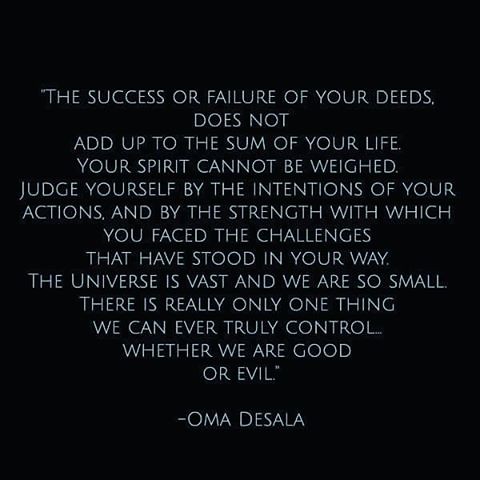In this image, against a solid black background, a profound quotation is presented in white text: “The success or failure of your deeds does not add up to the sum of your life. Your spirit cannot be weighed. Judge yourself by the intentions of your actions and by the strength with which you face the challenges that have stood in your way. The universe is vast and we are so small. There is really only one thing we can ever truly control: whether we are good or evil.” The quote is attributed to Oma Desala, with her name appearing below the text, also in white lettering.